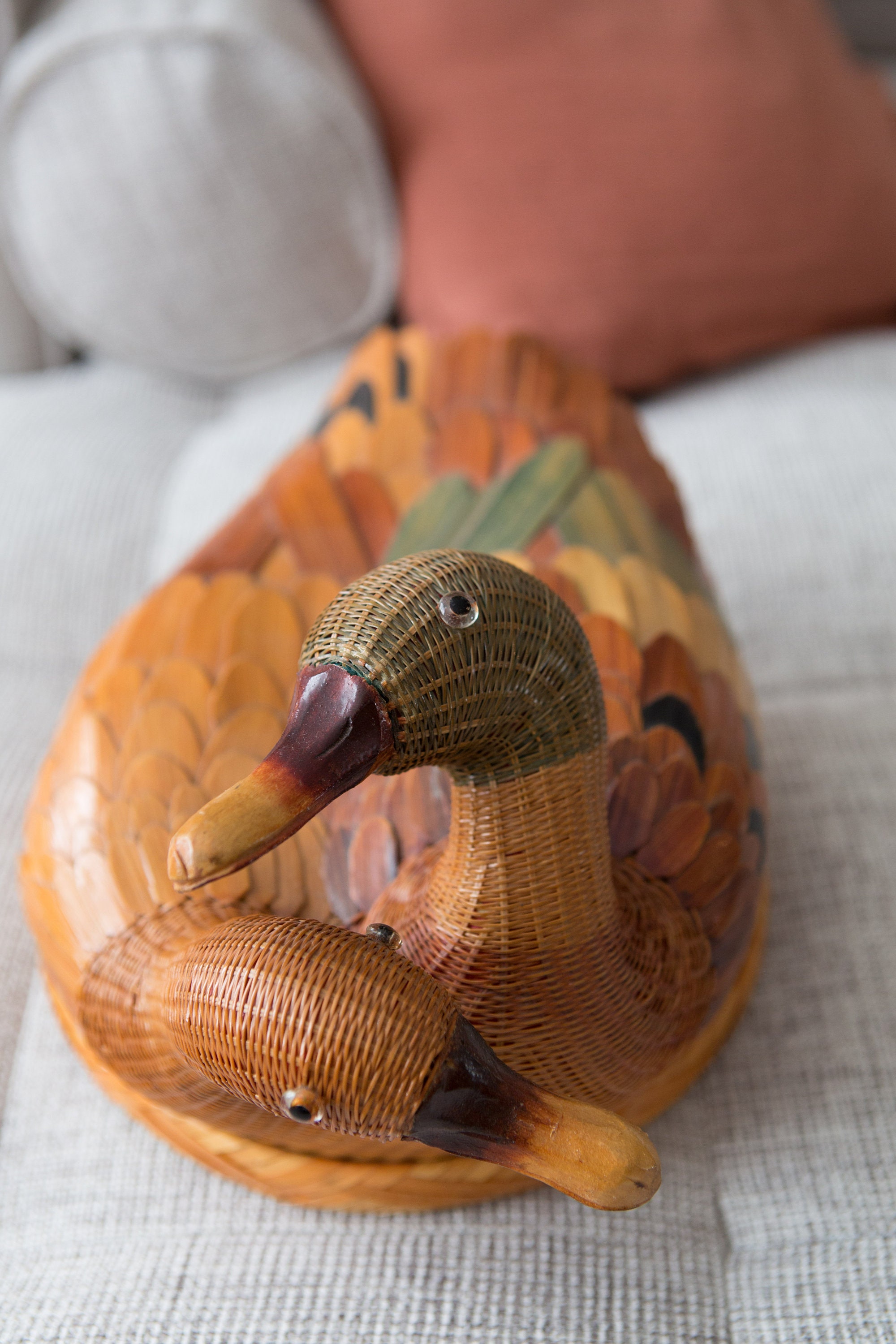This image features an intricately crafted wooden sculpture of a two-headed duck, blending artistry and realism. The two heads emerge from a single, ovate woven body that exhibits a sophisticated basket weave pattern. Each head showcases remarkable detail; the bills display gradient brown hues with the upper beak slightly darker, lending a striking, authentic appearance. The eyes seem to be delicately taped on, adding to the lifelike quality. The necks and feathers are meticulously carved and appropriately colored in various shades of brown, green, black, and tan, resembling a modern interpretation of natural duck plumage. The upper head, reminiscent of a mallard, has a grayish-green top, while the lower head rests just beneath it. Both are adorned with beautifully colored feathers that extend towards the back in greens and yellows for the upper head, and more browns for the lower. The sculpture is prominently positioned on a gray couch, complemented by decorative pillows, creating an elegant yet cozy backdrop.